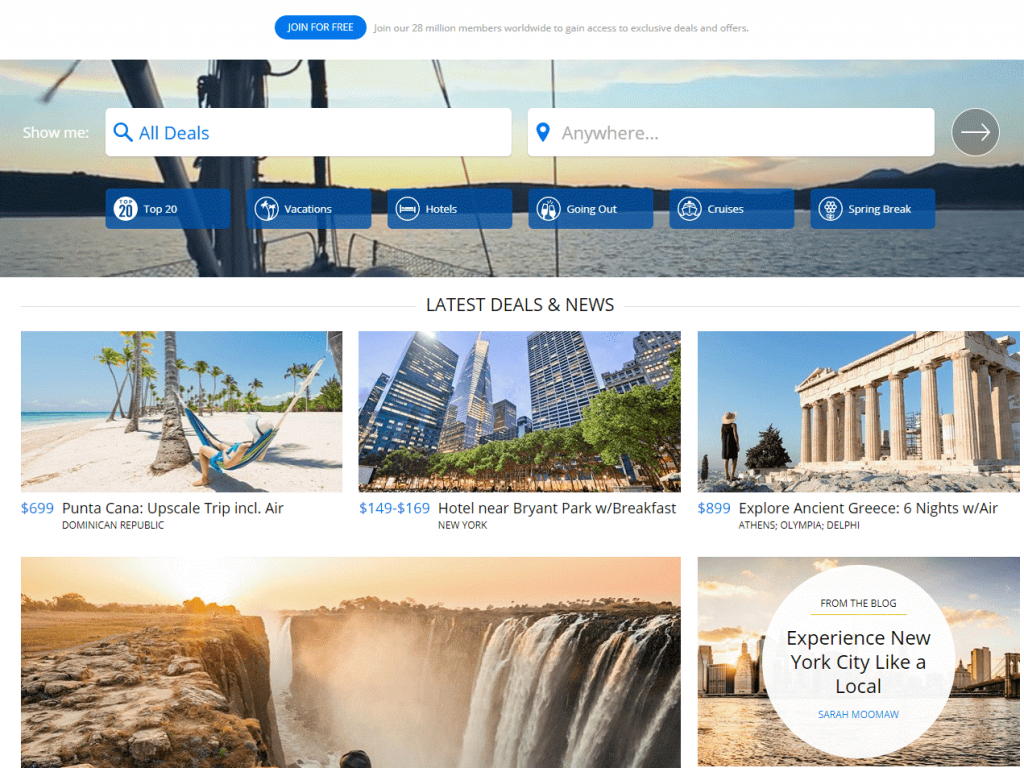This is an image of a travel deals website. At the top, there is a prominent "Join Here" button within a circle, inviting visitors to join 28 million members who have applied for access to exclusive deals and offers. While the company name is not displayed, the website highlights various deals.

In the background, there is a captivating image of a boat with its bow pointed towards the sea, framed by scenic, mountainous landscapes. The image features a soothing palette of blues and yellows.

Below the main image, there are several blue buttons labeled with categories such as "Vacations," "Hotels," "Going Out," "Cruises," and "Spring Break." Additionally, an "All Deals" button is visible along with a "Show Me" prompt where users can enter their information to receive the top 20 deals.

Further down, in the "Latest Deals and News" section, various offers are listed:

1. **Punta Cana** – $699, featuring an image of someone relaxing in a hammock.
2. **Hotel near Bryant Park with Breakfast, New York** – Prices range from $149 to $169.
3. **Explore Ancient Greece** – Six nights in Athens with airfare included, priced at $899.

Also displayed is an image of a large, unnamed waterfall, followed by a smaller square image promoting the experience of New York City like a local.

All these elements are visually organized to guide users through various exciting travel options and the latest deals available.